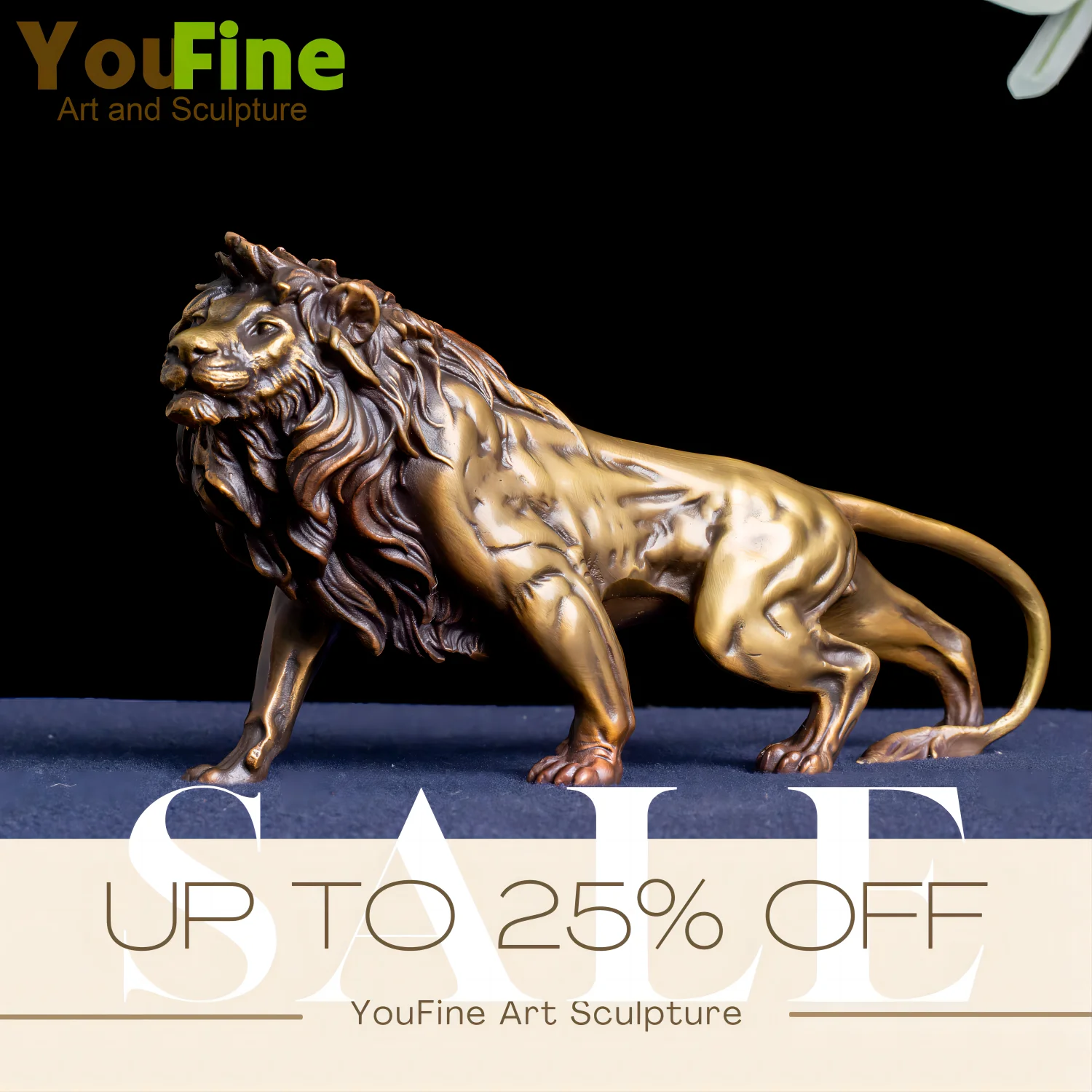This detailed advertisement from U Fine Art and Sculpture showcases a stunning bronze-gold lion statue as the centerpiece. The artwork, which could be produced by methods such as lost-wax casting but is not entirely confirmed, boasts intricate detailing, with finely rendered muscle definitions in the legs and carefully etched lines representing the flowing mane and facial features like the eyes and nose. The statue is set against a black background with a medium blue carpeted floor. The advertisement announces a sale of up to 25% off, prominently featured in the upper left corner amidst a deep black backdrop. The mention of "U Fine Art Sculpture" indicates the business's name, further highlighted by a mysterious floral element in the upper right corner, possibly petals. The overall composition suggests this advertisement would be fitting for a sophisticated fine art magazine.